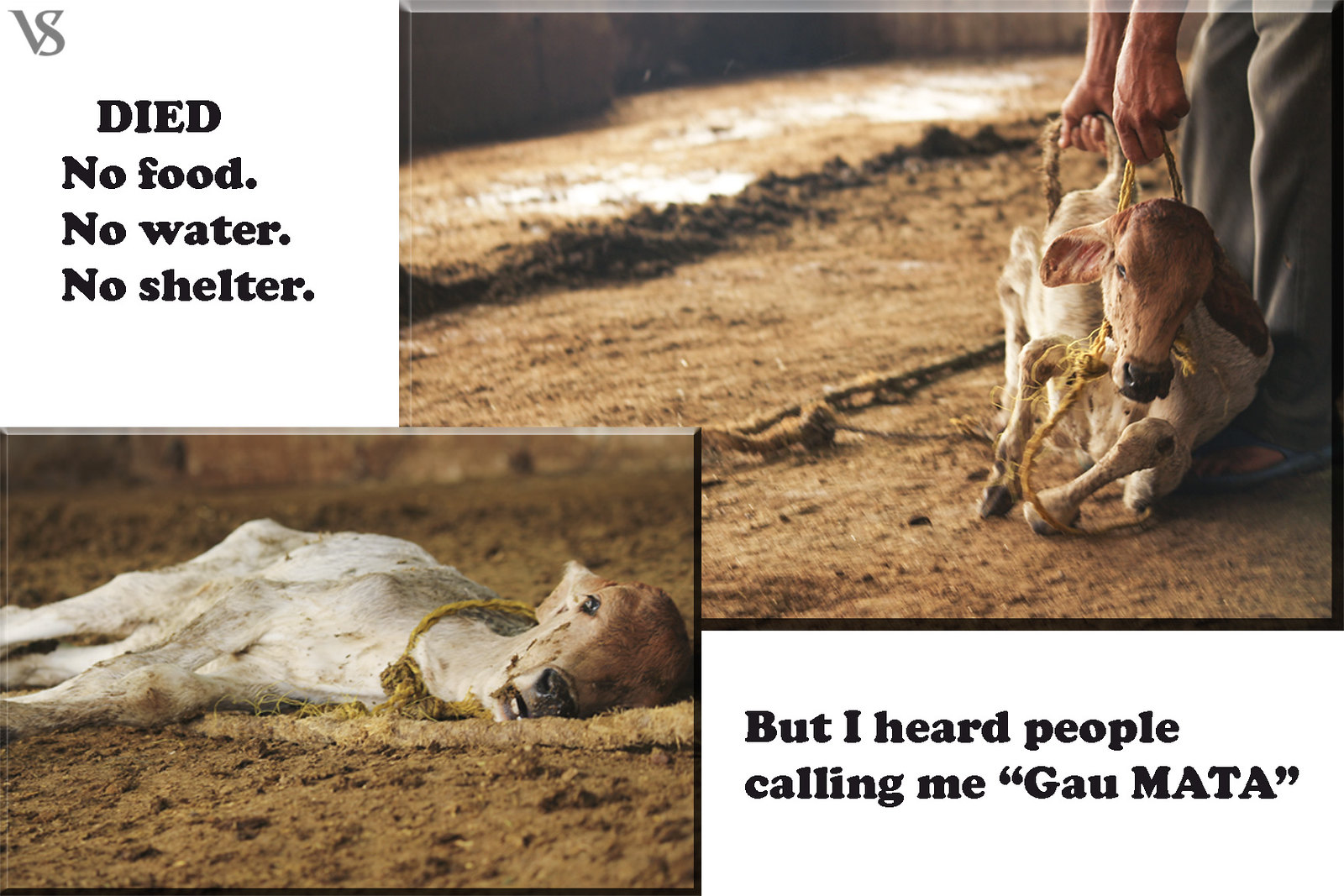The image appears to be a slide featuring a distressing scene of neglect involving a baby cow. In the upper left corner, there is a logo combining the letters "V" and "S." Below the logo, a black text reads, "Died. No food, no water, no shelter." The right side of the slide includes a photograph of a very skinny white and brown calf lying in the dirt with a yellow rope around its neck. A man's hands and feet, clad in light blue jeans, are seen pulling the rope, attempting to lift the calf. The left side of the slide shows another image of the same calf lying on its side in the dirt with its eyes open. The ground appears muddied with patches of hay. In the bottom right corner, black text in quotation marks states, "But I heard people calling me Gaumata."